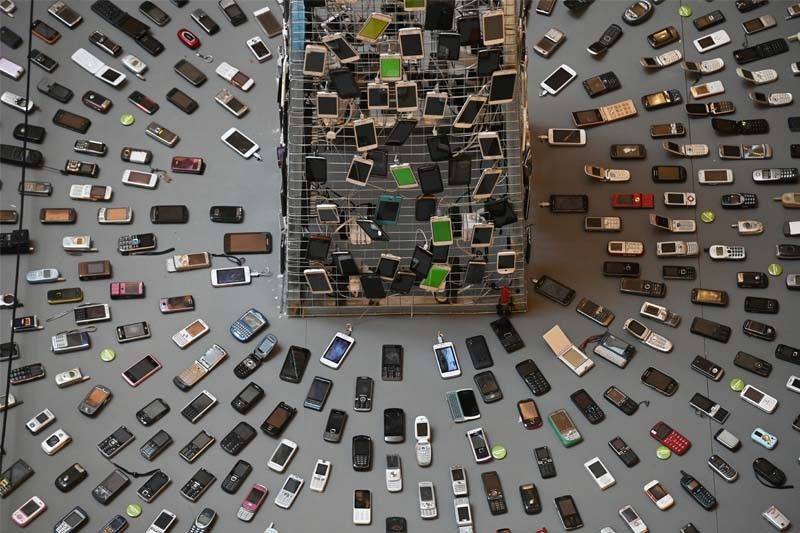This aerial photograph captures an intricate and detailed scene featuring dozens of cell phones of various ages and models, meticulously arranged in a circular pattern. At its core, the image reveals a central rectangular section filled with cell phones, either clipped on or attached via charging cables to a mesh or metal structure. Surrounding this central hub, the phones fan outwards in concentric circles, creating a visually striking sunburst effect. The outer circles showcase a diverse collection of phones pointing towards the center, including flip phones, old iPhones, Blackberries, slider phones, and even the occasional pebble phone. The arrangement displays a plethora of colors—from classic black, gray, and silver to standout shades like red, pink, and occasional green buttons. All the phones are turned off, with their screens or top faces directed towards the middle rack, set against a gray surface that might be a counter or floor. There is no text or written information within the image, emphasizing the striking visual tapestry of aging technology.